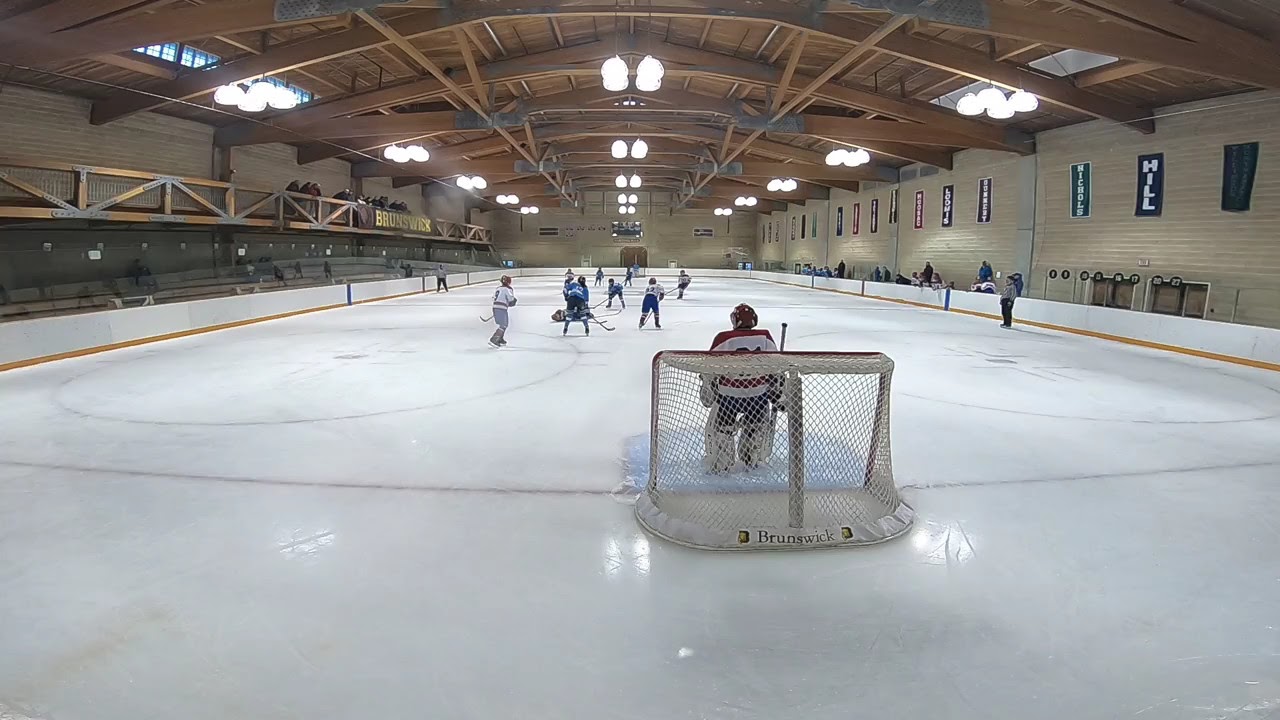The image captures an intense moment during an indoor ice hockey game, with a focal point slightly behind the goalie, providing a vantage point that showcases the action from just above the players' heads. The players are divided into teams wearing blue and white uniforms, with flashes of red accents, suggesting youth or young adult leagues. The goalie, dressed in a white jersey and helmet, wields his hockey stick determinedly while positioned in front of a white net branded with "Brunswick" at its base. The rink is lit by impressive, large hanging lights attached to substantial wood beams that arch across the ceiling, giving the space a sophisticated, non-gymnasium feel. On the right, a tan brick wall adorned with multicolored banners provides a backdrop. Referees flank both sides of the rink, and sparse spectators or possibly additional team members and coaches can be seen in the distance. The photograph, in color and landscape orientation, embodies a moment of photographic representational realism, capturing the essence of excitement and anticipation in a well-lit, modern indoor ice hockey arena.